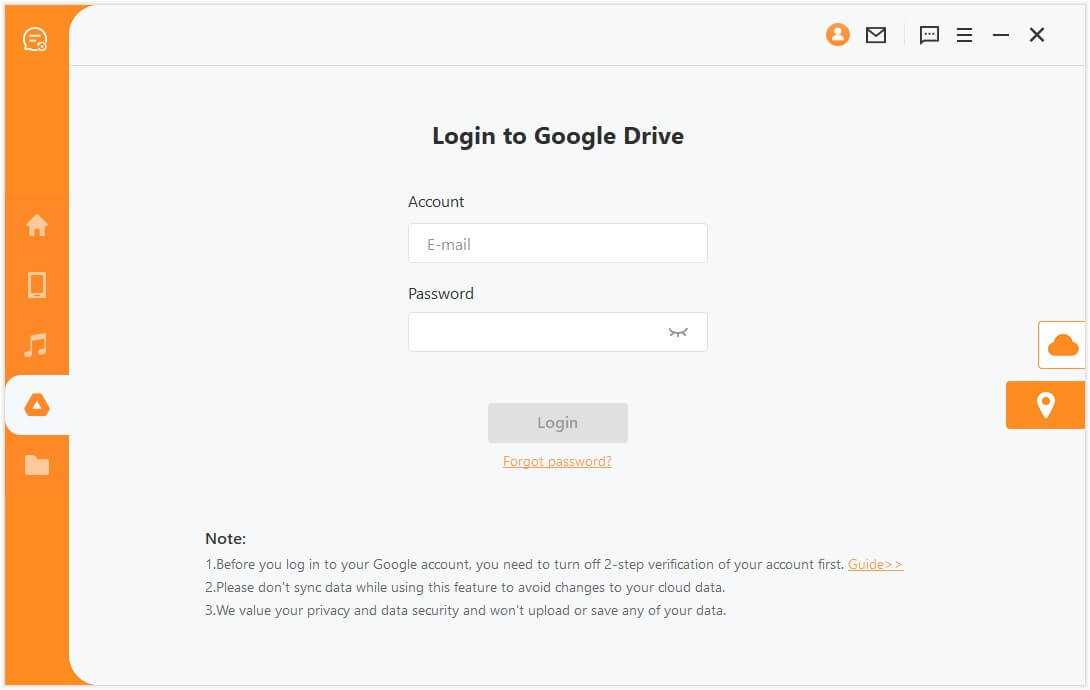The image depicts a login page for Google Drive. At the top, the header reads "Login to Google Drive." Below it, there are fields to input an email address and a password. A gray "Login" button sits beneath these fields, alongside an orange "Forgot Password" link.

Further down, there are three important notes outlined: 
1. "Before you log into your Google account, you need to turn off two-step verification of your account first." This note is accompanied by an orange "Guide" button that appears clickable.
2. "Please don't sync data while using this feature to avoid changes to your cloud data."
3. "We value your privacy and data security and won't upload or save any of your data."

On the right side of the page, there is a set of miscellaneous icons: a chat box, a home icon, a smartphone icon, a music note, and a files folder. 

At the top portion of the page, several distinct icons are visible:
- An orange circle with the outline of a person
- A mail icon
- A chat icon
- A line with black dots and a minus sign, likely for minimizing
- A black "X" for closing

The background of the page is predominantly white, with an orange sidebar adding a pop of color.